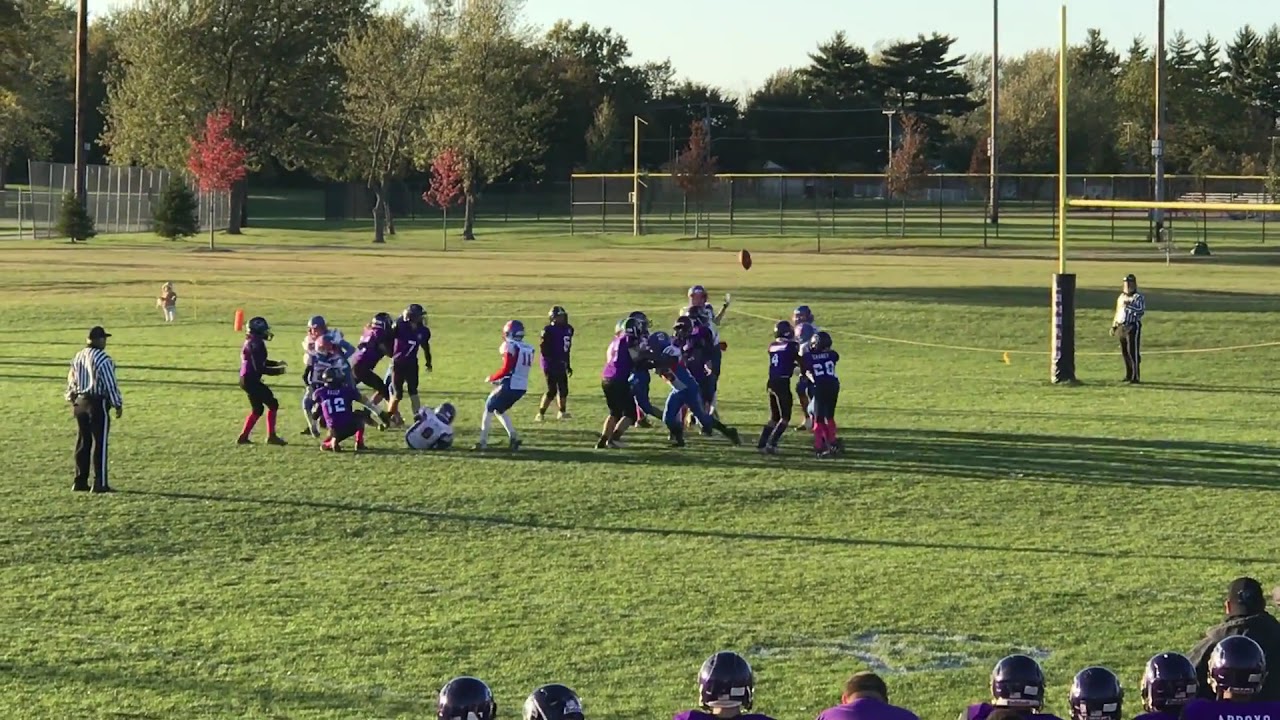This photograph captures a high school American football game in action on a large athletic field, which is prepared for multiple sports. Centered in the image, a football is suspended mid-air, just out of reach of a player in a white jersey who is attempting to catch it, indicating a moment of suspense in the play. The teams are distinguishable by their jerseys, one in dark navy and the other in light hues, with the players fully equipped in pads and helmets. 

In the foreground, about eight or nine team members, identifiable by their purple helmets, are seated on the sideline, watching the ongoing play intently. Among them sits an older man, likely the coach, without a helmet. Two referees, one on the left mid-range and another under the goalpost, closely observe the game, each wearing striped shirts and dark pants with stripes.

The background of the scene showcases a grass field extending into a schoolyard with distant tennis courts on the left and additional courts to the right. Scattered around the field are trees, some with red leaves and others with green, along with fences and electric light posts. The upper part of the image reveals a portion of the sky, pale blue and clear, adding to the picturesque outdoor setting.